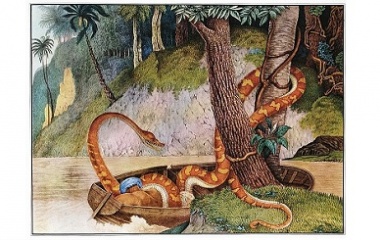This vibrant illustration depicts a dramatic scene set in a mountainous jungle by a murky brown river. Dominating the foreground is a long orange snake with yellow stripes coiled menacingly around a brown tree and extending its body onto a wooden boat. The snake appears to be guarding or attacking something within the boat, which also contains a blue tool. The boat seems precariously positioned near a small island, with waves gently lapping its sides, as if the snake is preventing the boat from drifting down the river. Surrounding this intense tableau are various kinds of trees, including lush palm trees, oak, birch, and a thick tree at the top right. The background features rugged, hilly mountains, enhancing the wild, untamed atmosphere of the scene, with a glimpse of the sky in the upper-left corner.